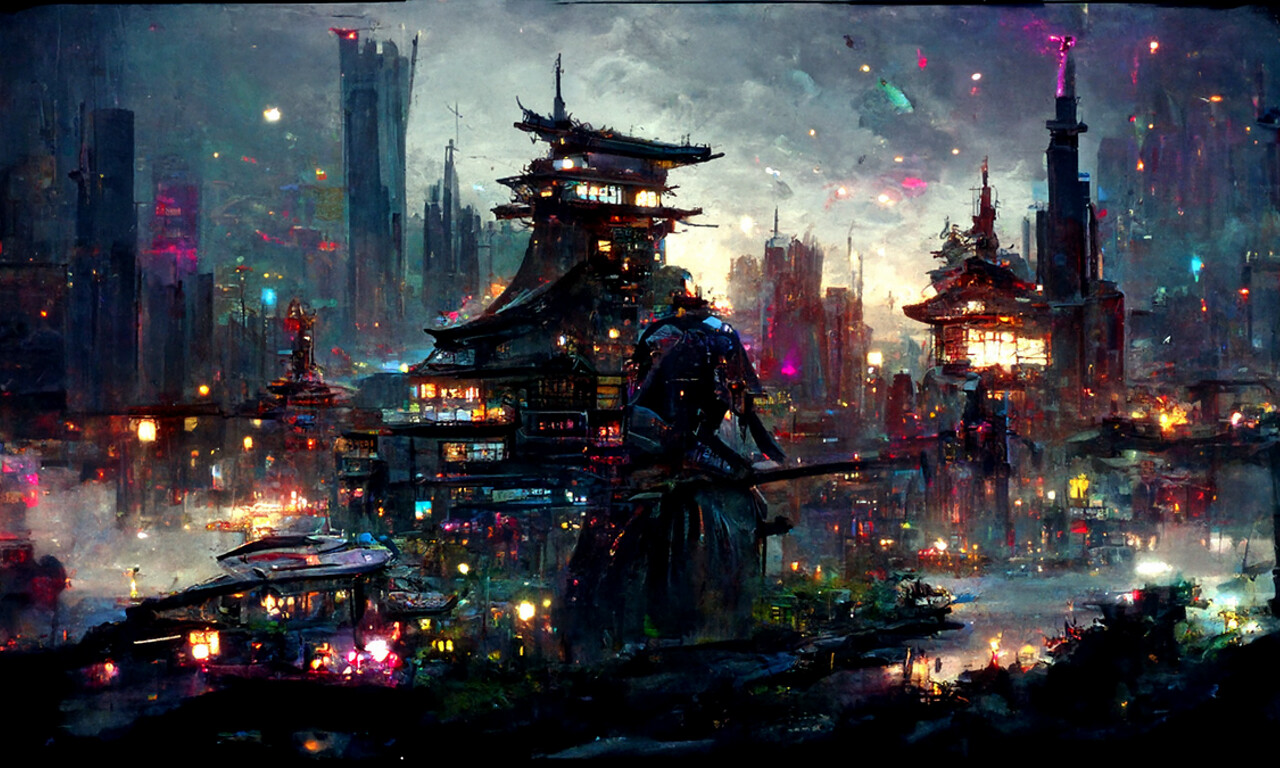This is a highly detailed and captivating landscape-oriented digital painting, evoking a cyberpunk and dystopian atmosphere with a blend of bright neon colors and dark, foreboding undertones. The scene is set in a futuristic city resembling traditional Japanese architecture, characterized by single-story buildings in the foreground and towering, ornate structures with sloped roofs in the background. Dominating the center of the image is a colossal, enigmatic robot, almost as tall as the surrounding buildings, ominously wielding a sword-like weapon. The sky is a mix of gray, scattered with bursts of light from the vibrant pink, green, blue, yellow, and magenta neon signs that illuminate the scene. The ground appears wet, reflecting the myriad of colors and lending a damp, somber mood to the setting. A waterway with several boats adds another layer of reflection and depth. The overall brushwork and texture suggest a vivid combination of oils or acrylics, enhancing the painting's rich and dynamic quality, making it an unforgettable representation of a dystopian, yet vividly imaginative, world.